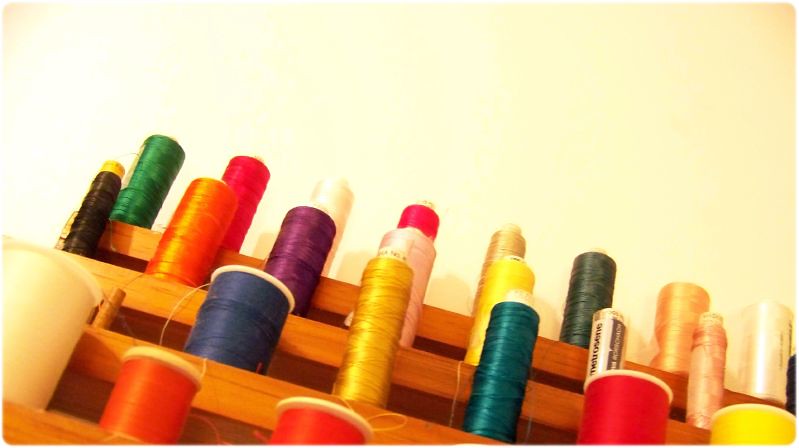The image depicts a neatly organized collection of variously sized spools of sewing thread, displayed on a light brown wooden shelf resembling a miniature staircase with four levels. The spools are tightly wound and come in a vast array of colors including bright green, pink, orange, purple, metallic purple, white, yellow, metallic yellow, red, black, tan, cream, and dark green. Each spool is placed on its own spindle, secured by a small knob in the middle of the shelf's steps. The spools vary in dimensions, with some being shorter and thicker, while others are taller and more slender. The wooden spool holder, which facilitates this structured arrangement, sits against a plain white wall background, highlighting the vivid hues of the thread.